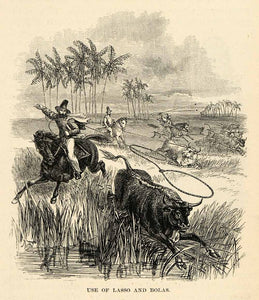This historical scene, resembling an old print in a book, depicts a vivid portrayal of cowboys wrangling cattle, seemingly set in a tropical or marsh-like landscape characterized by palm trees and tall grass. The central focus is a black bull about to be lassoed by a cowboy on a galloping black horse. The intricate detail, especially in the foreground, highlights the period attire and tack, possibly from the 1700s. In the background, additional riders are seen attempting to lasso other bulls, with lighter-colored animals dotting the scenery. The drawing, on what appears to be aged paper with a beige tint, features the inscription "Use of Lasso and perhaps Bowler or Dollar," adding a historical context to the detailed, dynamic action in the scene.